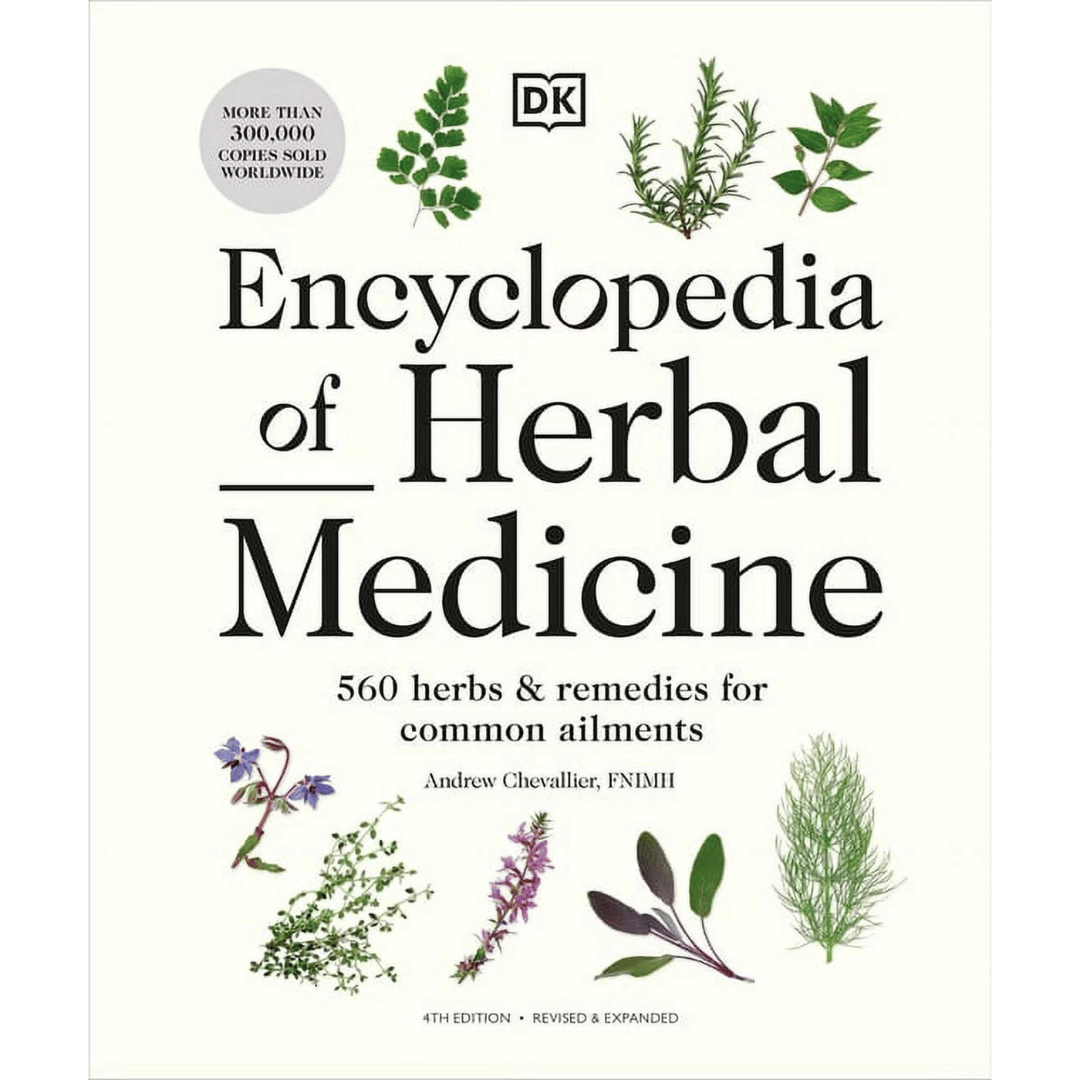The cover of this book, "Encyclopedia of Herbal Medicine," features an ivory white background adorned with illustrations of various plants and herbs, showcasing hues of green, purple, and blue. Prominently displayed in the center, the title "Encyclopedia of Herbal Medicine" is written in bold black text, followed by the subtitle "560 Herbs and Remedies for Common Ailments." The author, Andrew Chevalier, F-N-I-M-H, is listed underneath. At the top left corner, a gray circle highlights that over 300,000 copies have been sold worldwide, and nearby, the logo "DK" appears in the form of a small book. The bottom of the cover denotes that this is the Fourth Edition, Revised and Expanded, emphasizing its enriched content. The entire cover is framed with detailed botanical illustrations, indicating the comprehensive nature of the herbal knowledge contained within.